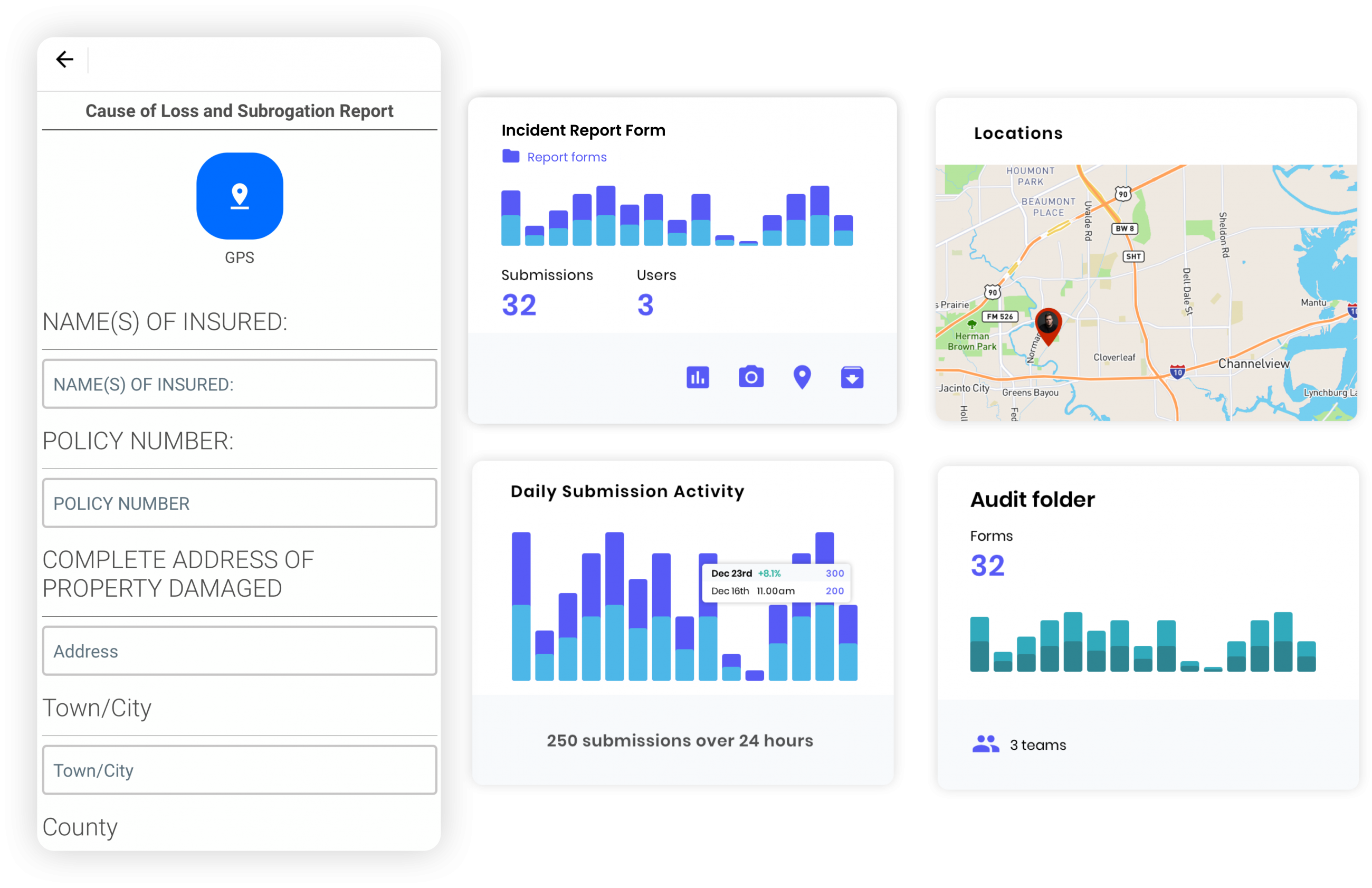Detailed Caption:

The image presents a side-by-side comparison of a mobile interface and a series of graphical elements. On the left, there is a screenshot of a smartphone displaying a form titled "Cause of Loss and Subrogation Report." Prominently, a small blue square with a GPS icon and location symbol is visible, suggesting location-based data entry. The form includes various fields such as "Name of Insured," "Policy Number," "Complete Address of Property," "Town and City," and "Country," each accompanied by rectangular input boxes for user entry.

To the right of this mobile interface, there are four distinct graphical elements arranged in a 2x2 grid. The top left and bottom left panels each show bar graphs composed of teal turquoise at the bottom transitioning to a darker purple-blue at the top. Both graphs display a pattern of peaks and valleys, indicating fluctuating data trends. The bottom right graph mirrors this pattern but utilizes a color scheme transitioning from darker green at the base to the same teal turquoise higher up. Lastly, the top right panel features a map akin to a digital map application, marked with a noticeable red location pin, indicating a specific geolocation.